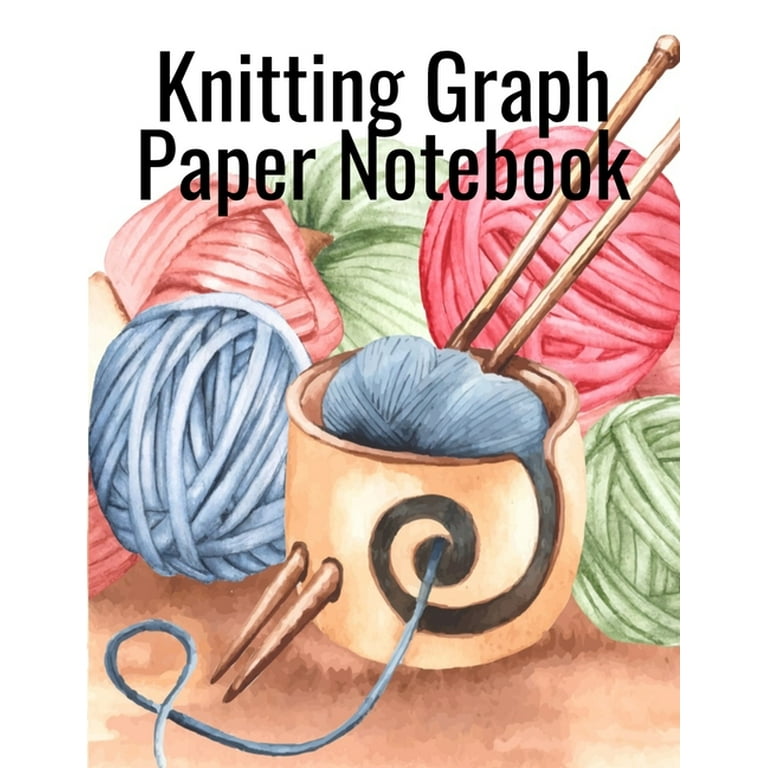The image features the cover of a "Knitting Graph Paper Notebook," prominently displayed in bold black lettering across the top against a white background. The central illustration, possibly done in colored pencil, showcases a vibrant array of yarn balls arranged on what appears to be a brownish table. There are five distinct balls of yarn in total: an orange, a green, and a pink ball aligned to the right, with a large blue ball in front of them. Centrally positioned is a golden cup adorned with a black swirl design and two holes at its base, through which two knitting needles are threaded. This cup contains another blue ball of yarn, with strands extending outwards and artistically curling around the cup. To the right of the cup, a partial green yarn ball is visible. The overall composition is colorful and inviting, setting a creative tone for the knitting-themed notebook.